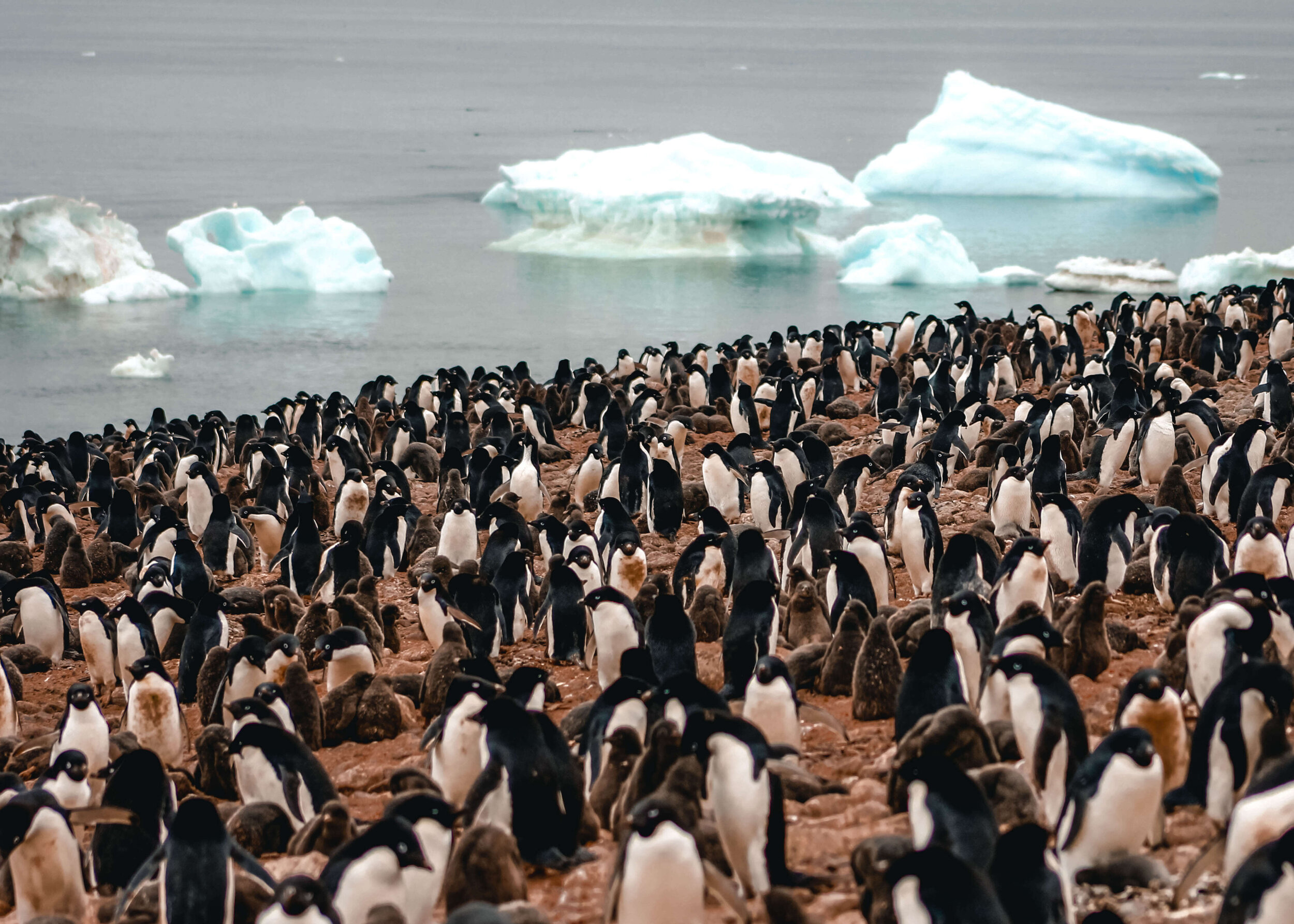The photograph captures a vast colony of penguins occupying a flat, rocky expanse that stretches across the bottom two-thirds of the image. The adult penguins, characterized by their white stomachs, black backs, and small pointed orange beaks, stand among their shorter, fuzzier black-feathered chicks. The land beneath them is a rugged brown surface, dotted with dense clusters of birds as far as the eye can see. Towards the top half of the image, a large body of blue water is visible, interspersed with several chunks of ice ranging from white and brown to a light blue hue. The shoreline curves upward from left to right, separating the packed penguins on land from the serene yet icy waters. There appears to be a few brown animals, possibly seals, among the penguins on the bottom left and just right of the center. The scene, bathed in daylight, suggests a natural habitat likely located in the Southern Hemisphere. This detailed depiction highlights the daily life of penguins in their natural environment, with the contrasting elements of land and ice present in this vibrant ecosystem.